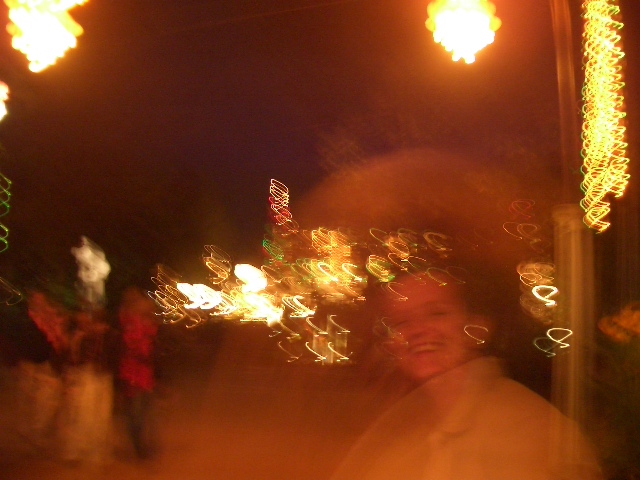In this night-time photograph, the scene is dominated by a single individual in the foreground, whose face is the clearest element in an otherwise blurry composition. The person, positioned centrally, is smiling, revealing the upper row of teeth, and has a brownish shading above their head. The background is significantly out of focus, containing three indistinct figures who appear to be socializing. The image is punctuated with various blurry lights, including circular lights with squiggly lines emanating from them, situated to the right. Additionally, a vertical sequence of yellow squiggly lines is visible in the upper right corner, adjacent to a bright white and yellow light. The left upper corner also features a similar bright light. The rest of the background remains enveloped in darkness, contributing to the photograph’s nighttime ambiance.